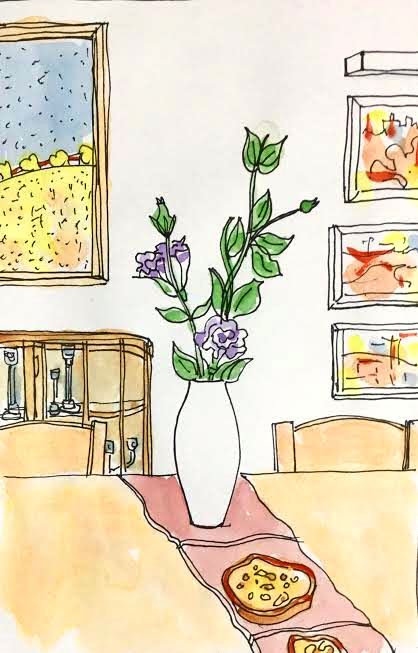The image is an artistic pen-and-ink style illustration, enhanced with watercolor fills that give it a soft and textured look. It depicts a cozy dining area. On the left, a brown wooden framed painting hangs on a white wall, showcasing a serene scene of a blue sky and a yellow field, which might have small bushes and a fence in the foreground. Below the painting, there's a small brown wooden china cabinet with glass doors that contain what looks like candlesticks.

Central to the image is a tan-colored table adorned with a pale pink runner, positioned diagonally, upon which sit two pizzas. Two matching tan chairs are pushed in against the far side of the table. At the edge of the table's center, there is a tall white vase holding a plant with long yellow leaves and delicate purple frilly flowers.

On the right side of the wall, three vertically aligned rectangular paintings dominate the space, exhibiting vibrant hues of red, orange, and yellow, illuminated by a picture light that adds focus and warmth to the artwork. The scene is a loose yet detailed watercolor sketch, balancing between abstract impressions and realistic elements, predominantly using brown, purple, and neutral tones. The overall composition captures a whimsical yet grounded moment within an inviting dining space.